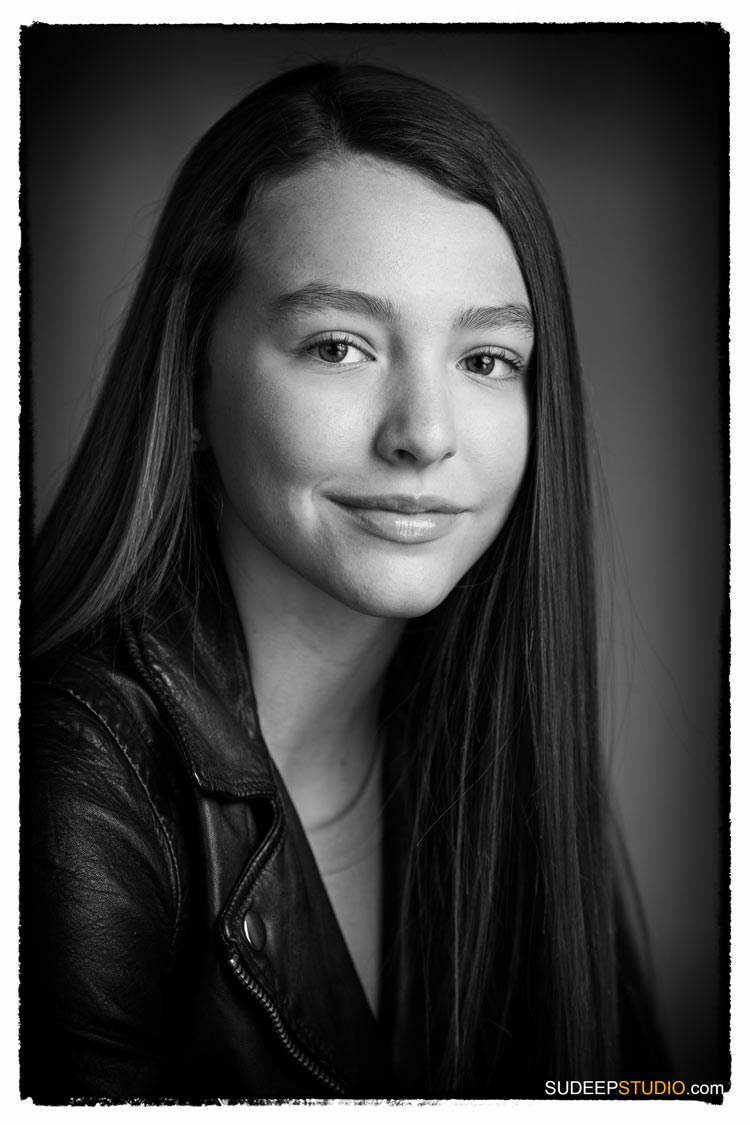This is a black-and-white headshot of a young woman in her mid-twenties with a distinctive heart-shaped face, thick lips, and a slight dimple on her right cheek. She has long, straight hair, likely brown, parted to the side and left unclipped. Her skin appears fair. She is adorned in a black leather jacket featuring wide lapels that gape open at the front, revealing the neckline of a lighter-colored t-shirt beneath. Metal accents on the jacket, including a silver zipper and a button, add to the details. The background is a rich charcoal gray with white shading near her head, giving the impression of a worn, crinkled photograph. Her expression is a subtle, becoming half-smile that exudes a confident and slightly playful demeanor. In the bottom right-hand corner of the image, "SudeepStudio.com" is printed, with "Sudeep" and ".com" in white and "Studio" in yellow.